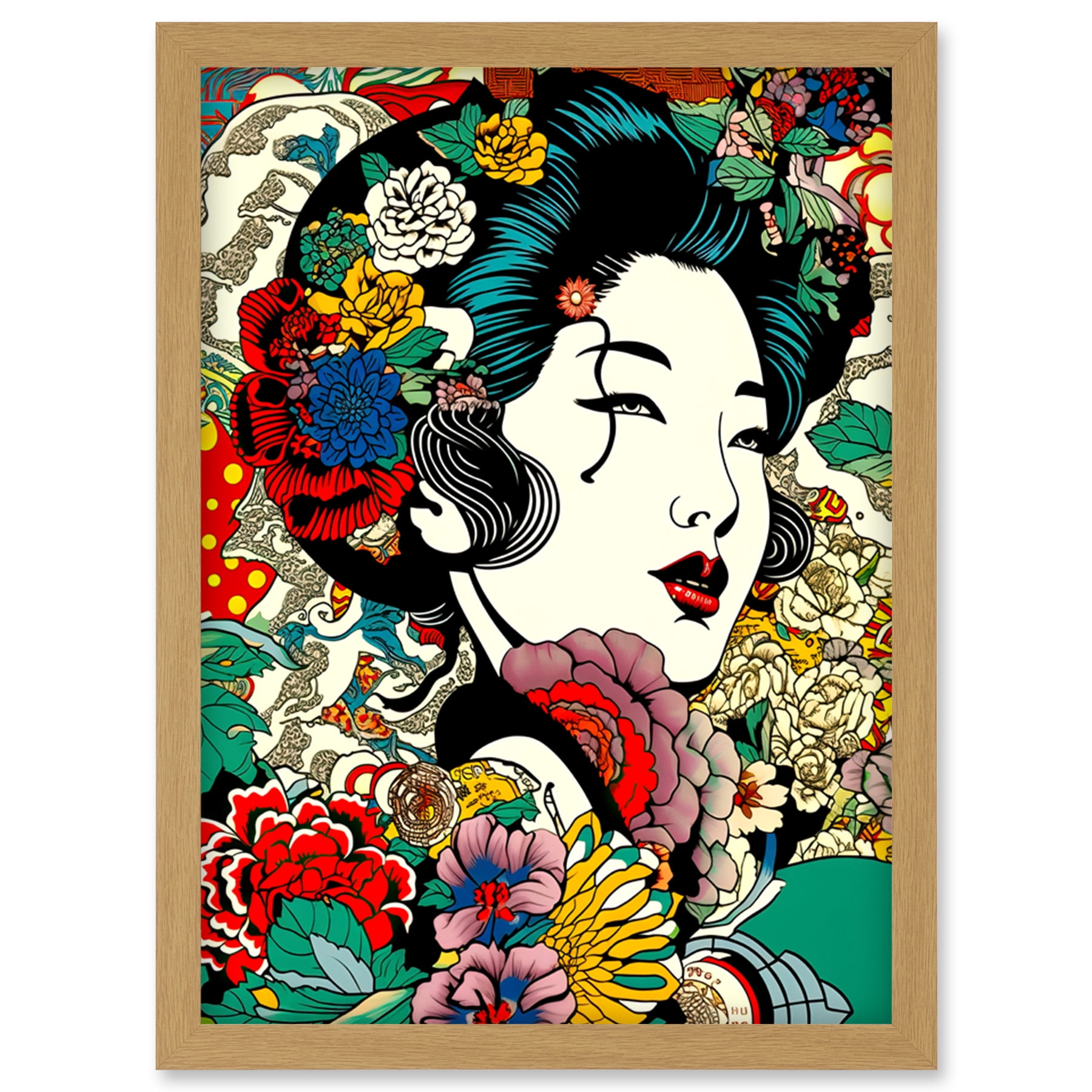This vibrant and detailed portrait appears to be a computer-generated or digitally painted image of an Asian woman, likely representing a traditional geisha. She has pale skin and striking red lipstick that accentuates her serious expression as she gazes into the distance. Her voluminous black hair, styled up, is adorned with a multitude of colorful flowers, including yellow, white, blue, and red blossoms, with a strand cleverly positioned across her right cheek. The background and her outfit are engulfed in an array of vividly colored flowers and artifacts, featuring colors such as orange, yellow, green, blue, brown, and beige. Intricate patterns, including polka dots, stripes, and leopard prints, add depth and texture to the scene, evoking an oriental design. The entire picture is beautifully framed in a wooden frame, enhancing its traditional yet vibrant aesthetic.